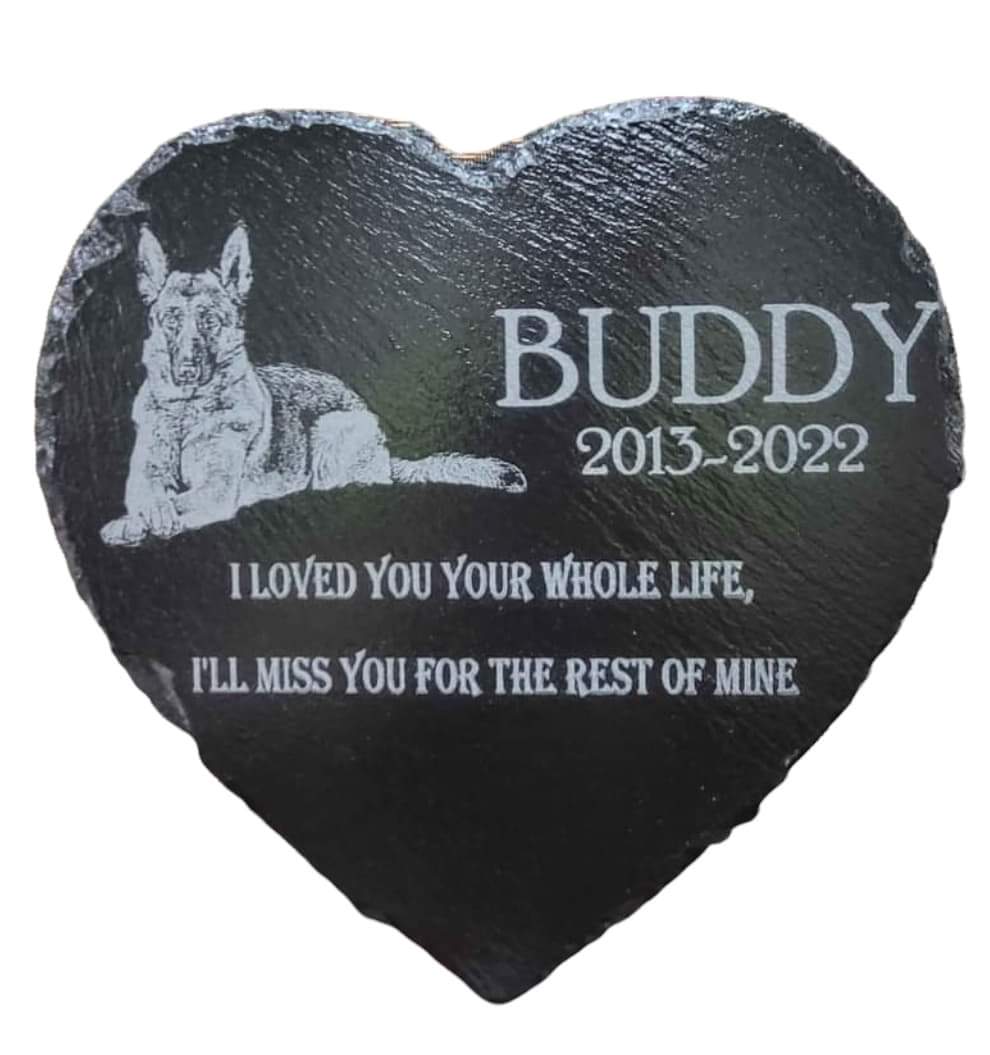The image depicts a heart-shaped concrete memorial for a German Shepherd named Buddy, who lived from 2013 to 2022. The heart is painted in a shiny black finish and features a detailed gray illustration of Buddy, with notes of bluish gray. The dog is depicted with defined features such as a well-drawn nose, eyes, and ears, as well as a black tuft at the end of its tail and black fur along its back. Buddy's name appears in bold capital letters near the image, with a unique font where certain letters like V, Y, and W have an extra lift on the right part of the top of the letter and a slight shadow effect. Below the image and name, the text reads: "I loved you your whole life. I'll miss you for the rest of mine." This touching caption underscores the sentiment of the memorial. The design is rough-edged, adding a raw and heartfelt quality to the tribute.